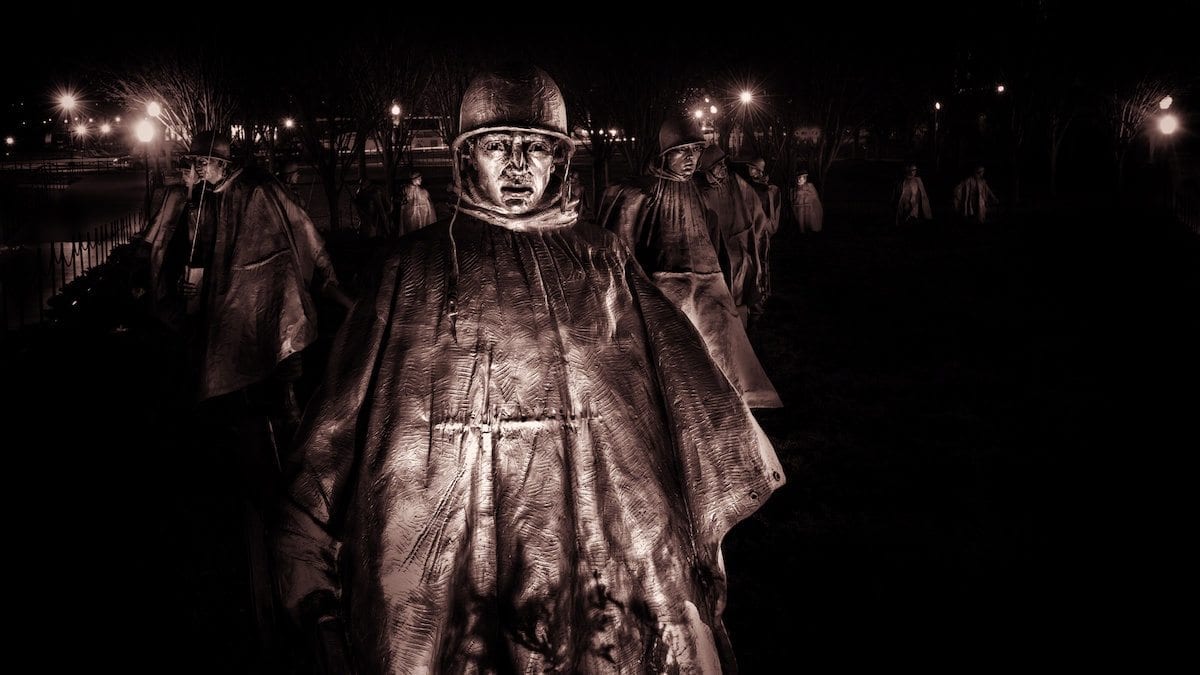The black and white nighttime photograph depicts a dramatic and somewhat eerie scene featuring a sculptural exhibit of soldiers. The background is enveloped in darkness, punctuated by glowing streetlights that create a halo effect, enhancing the starburst appearance of the light. Four soldiers stand prominently in the foreground, their figures steadfast in raincoat-like robes and helmets, suggesting historical military attire—possibly from a past war such as the Civil War or World Wars. The figures stretch into the background with more similarly dressed soldiers to the left and right. The stark contrast of blacks, dark grays, and whites, alongside the intricate shadows and highlights, creates a hauntingly realistic effect that initially makes the statues appear as real men. A small, indistinguishable building can be observed faintly in the background, adding to the overall mysterious and somber atmosphere of the image.